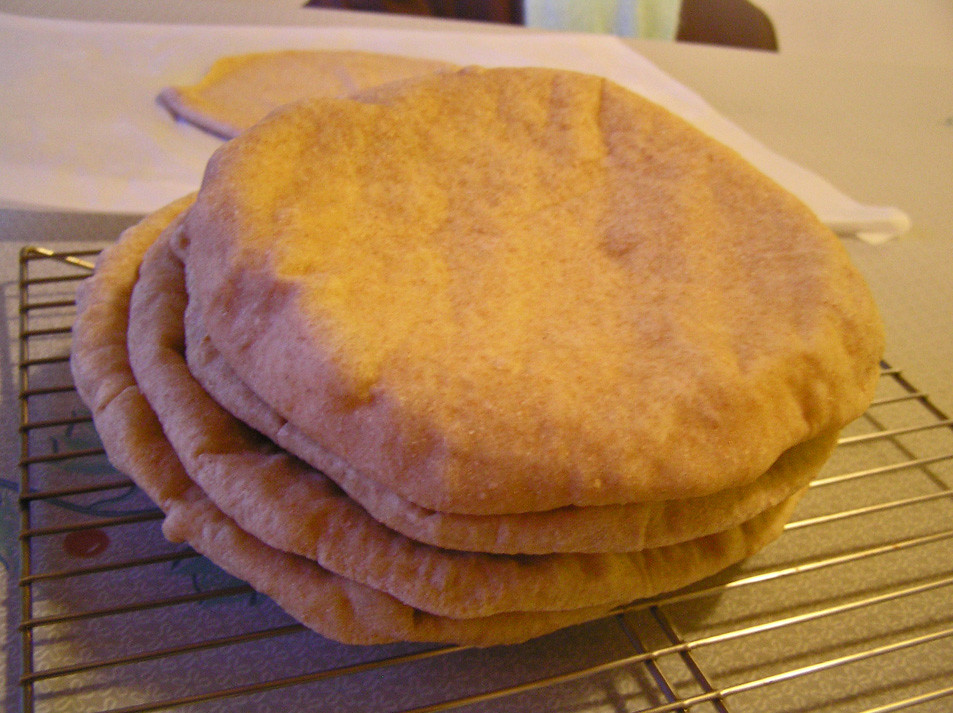The image depicts a low-light scene of a tan-colored countertop adorned with a delicate, embroidered cloth featuring green leaves and a red berry on the left-hand side. Atop this cloth sits a wire cooling rack with closely spaced bars, holding four golden-brown, whole wheat pita breads stacked neatly on top of each other. The homemade quality of the pitas is suggested by the presence of rolled-out dough, partially visible on what appears to be wax paper or parchment paper in the background. A white napkin or paper towel also lies in the background, with another single piece of pita bread resting upon it, illuminated by a warm, yellowish incandescent light that adds a cozy ambiance to the grainy photo.